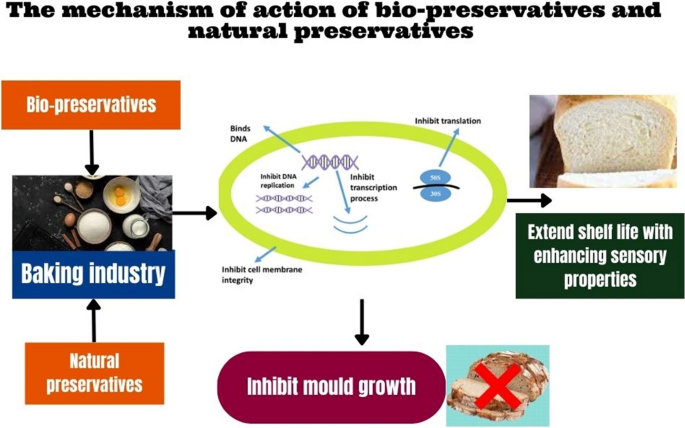The image is a detailed flowchart set against a white background, illustrating the mechanism of action of biopreservatives and natural preservatives. At the top is a bold black text title: "The Mechanism of Action of Biopreservatives and Natural Preservatives." Below it, in the top left, there's an orange rectangular box labeled "Biopreservatives" in white text. An arrow points down to an image depicting common baking ingredients such as flour, eggs in a bowl, a pitcher of milk, spoons, cinnamon sticks, all on a black background. Below this image, it says "Baking Industry" in white text on a blue background.

An arrow points up from the "Baking Industry" box to another orange box labeled "Natural Preservatives" in white text. From the "Baking Industry" box, a black arrow points right to a green oval with a white center, surrounded by various mechanistic descriptions. The green oval has an arrow pointing left and is labeled "Inhibit Cell Membrane Integrity."

Inside the white center of the oval, there's a DNA graphic with multiple interconnected arrows and texts describing the preservation mechanisms. To the top left, an arrow labeled "Inhibit DNA Replication" points down diagonally. The central DNA strand has an outward arrow that reads "Binds DNA." Below, another arrow points down to "Inhibit Transcription Process." Two additional blue-grey ovals further connect to a "Inhibit Translation" label.

An arrow from the bottom of the green oval points to a capsule-shaped box labeled "Inhibit Mold Growth." To the immediate right of this box, there's an image of moldy bread marked with a red X. Another arrow from this section points up to a green rectangular box that says "Extend Shelf Life by Enhancing Sensory Properties" in white text, with an image of sliced white bread positioned above.

This comprehensive flowchart visually explains how biopreservatives and natural preservatives interact to improve the shelf life and sensory properties of baking goods while inhibiting mold growth and affecting various cellular processes.